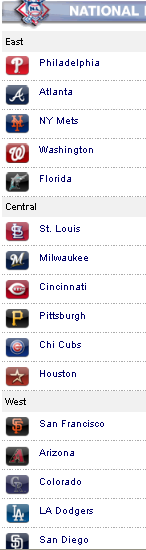The image is a screenshot displaying a vertical list taken from a website. The screenshot is somewhat low-quality, with a noticeable blur and pixelation. At the top of the screenshot, there's a bluish bar with white text that reads "National," accompanied by an icon resembling a circle with two hockey sticks. 

Below the blue bar, there is a gray rectangle with the word "East" in black text, followed by a list of Eastern baseball teams. The listed teams include Philadelphia, Atlanta, New York Mets, Washington, and Florida, each with their respective team logos positioned to the left of their names. 

Next, another gray rectangle with the word "Central" in black text introduces the Central division's teams. The teams listed here are St. Louis, Milwaukee, Cincinnati, Pittsburgh, Chi Cubs, and Houston, all accompanied by their team logos to the left.

Further down, a gray rectangle with the word "West" in black text heads the section for Western teams. The teams listed under this category are San Francisco, Arizona, Colorado, LA Dodgers, and San Diego, each also featuring their respective team logos to the left.

The overall structure and content suggest that this might be a segment from a fantasy baseball website or a sports portal listing teams by division.